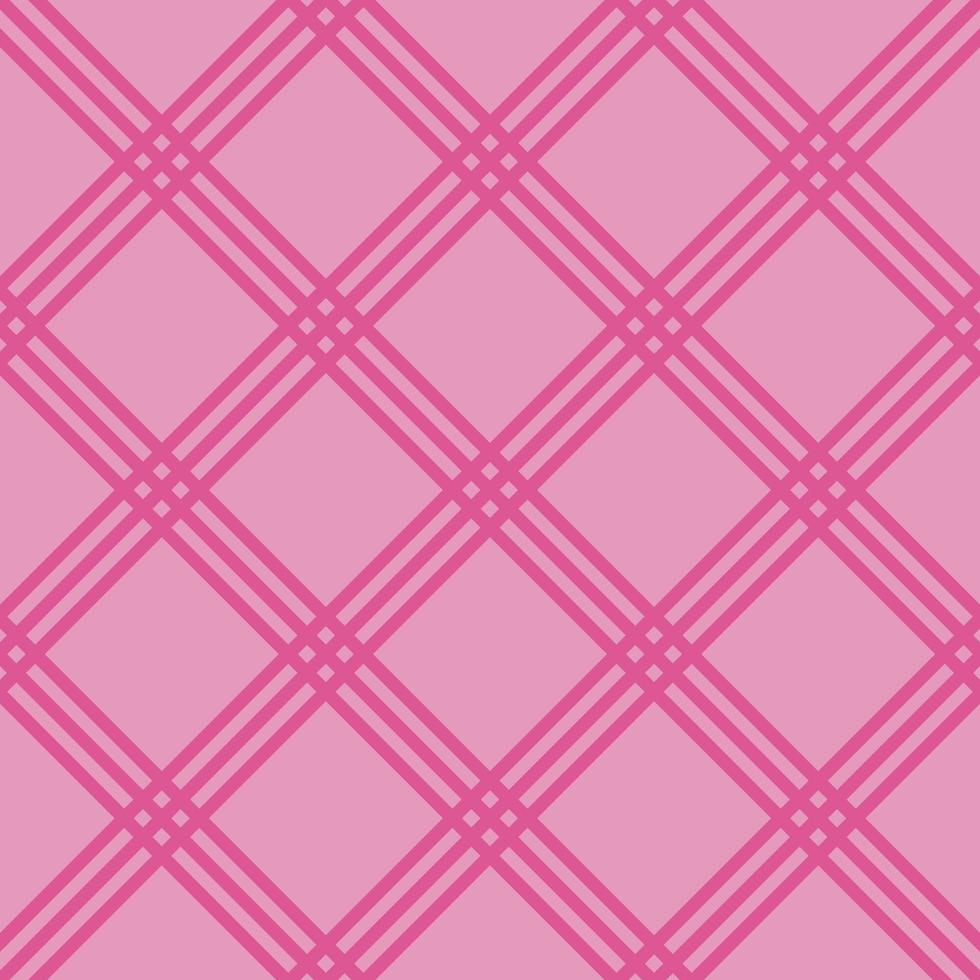This illustration features a seamless, repeating tartan pattern characterized by an intricate crisscross design. The background is a light pink hue over which three darker, almost hot pink lines intersect horizontally, vertically, and diagonally. This intersection forms prominent X shapes that repeat consistently across the design. The X shapes create diamond patterns, which further subdivide into even smaller diamond and square elements where the lines meet perpendicularly. The pattern, reminiscent of a picnic grid or wrapping paper, evokes a classic tartan look with its simple yet visually engaging geometric structure, making it suitable for backgrounds, wallpapers, or fabric designs.